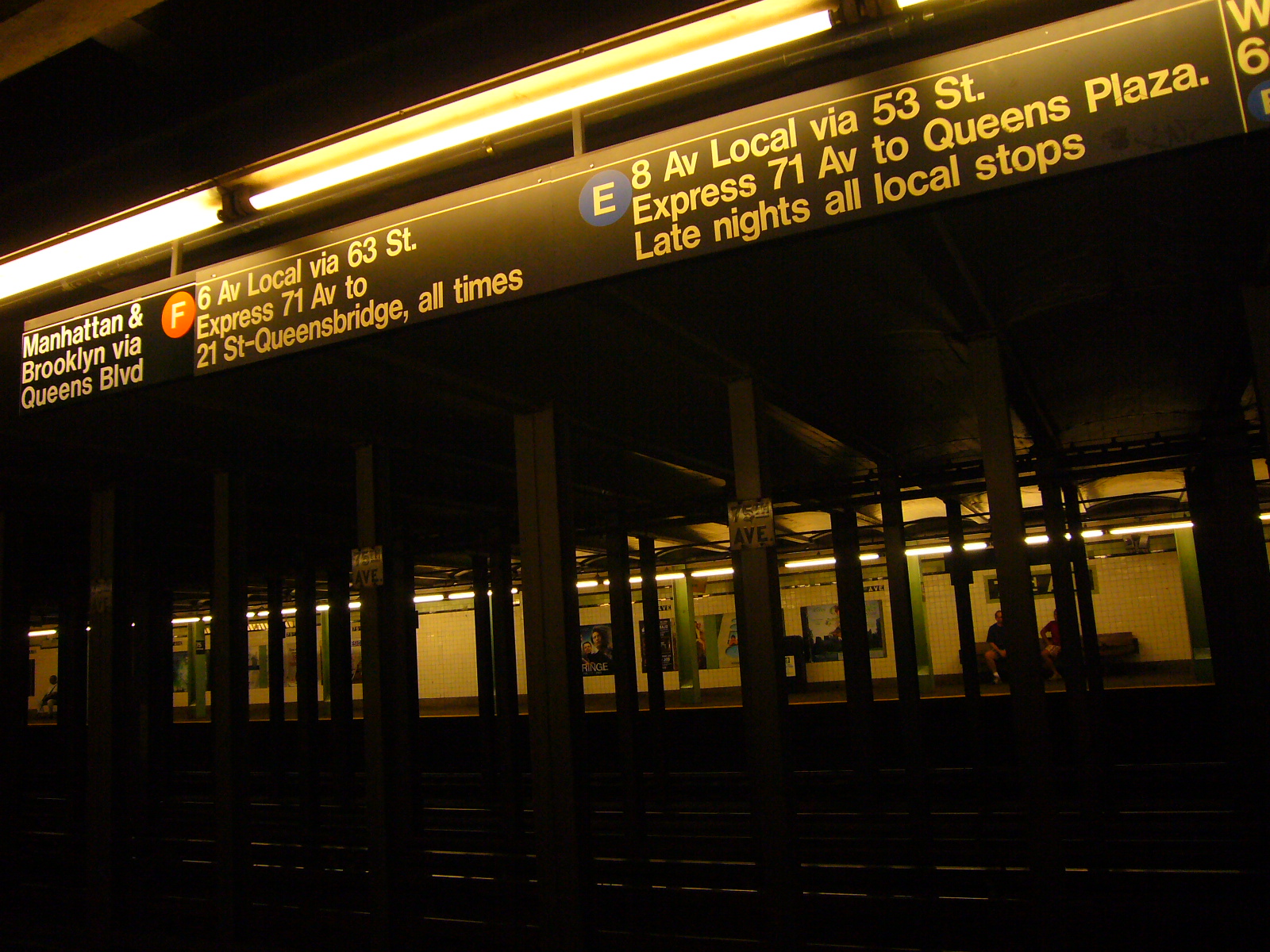The photo captures a dimly lit, underground subway station at night, showcasing an empty subway car. Bright fluorescent lights illuminate the signs above, which indicate various routes: "Manhattan and Brooklyn via Queens Blvd," "F, 6 Avenue Local Express," and "E, 8 Avenue Local Express to Queens Plaza, late nights, all local stops." The station features yellow-tinged walls due to the bright lighting behind the subway. A discreet figure leans against a wall adorned with photos, adding a solitary human element to the otherwise quiet, eerie environment. The overall atmosphere suggests a desolate, late-night setting in a bustling metropolitan transit system.